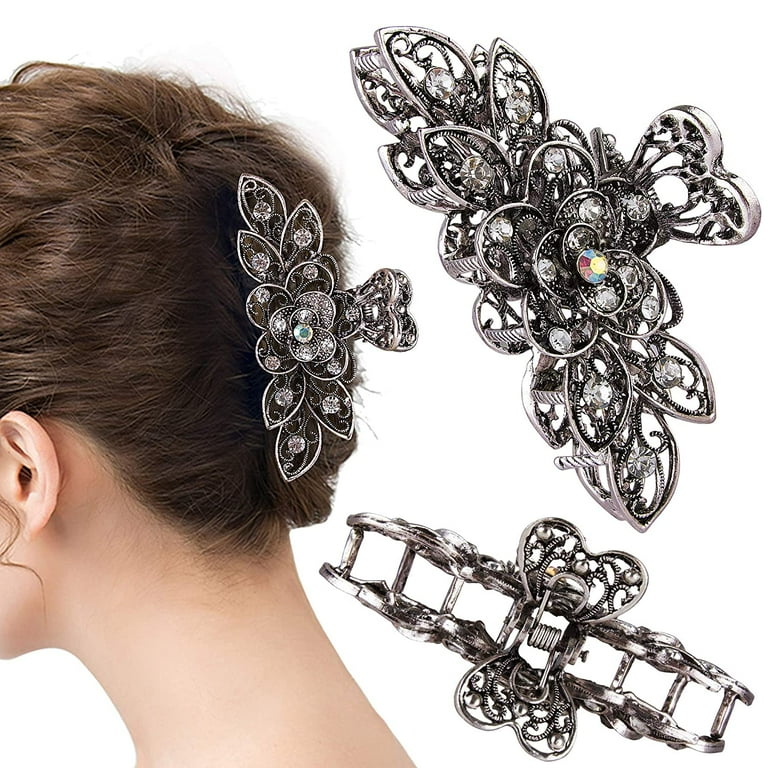The image showcases an ornate, silver hair clip from two angles: one from the front and one from the back. The front view, positioned at the top right, reveals the elaborate design—a leaf-like pattern with a colorful round pebble in the center. Surrounding this centerpiece, the clip features clear, diamond-like studs embellishing its petal and leaf motifs, giving it a sparkling, floral appearance. The mechanism of the clip is visible in the bottom right, displaying its intricate construction. On the left side of the image, the back of a woman's head with dark brown hair is visible. The hair is gathered and secured by the decorative clip, offering a clear view of its placement and ornamental detail. The background is white, providing a stark contrast that highlights both the woman's hair and the elegant hair accessory.